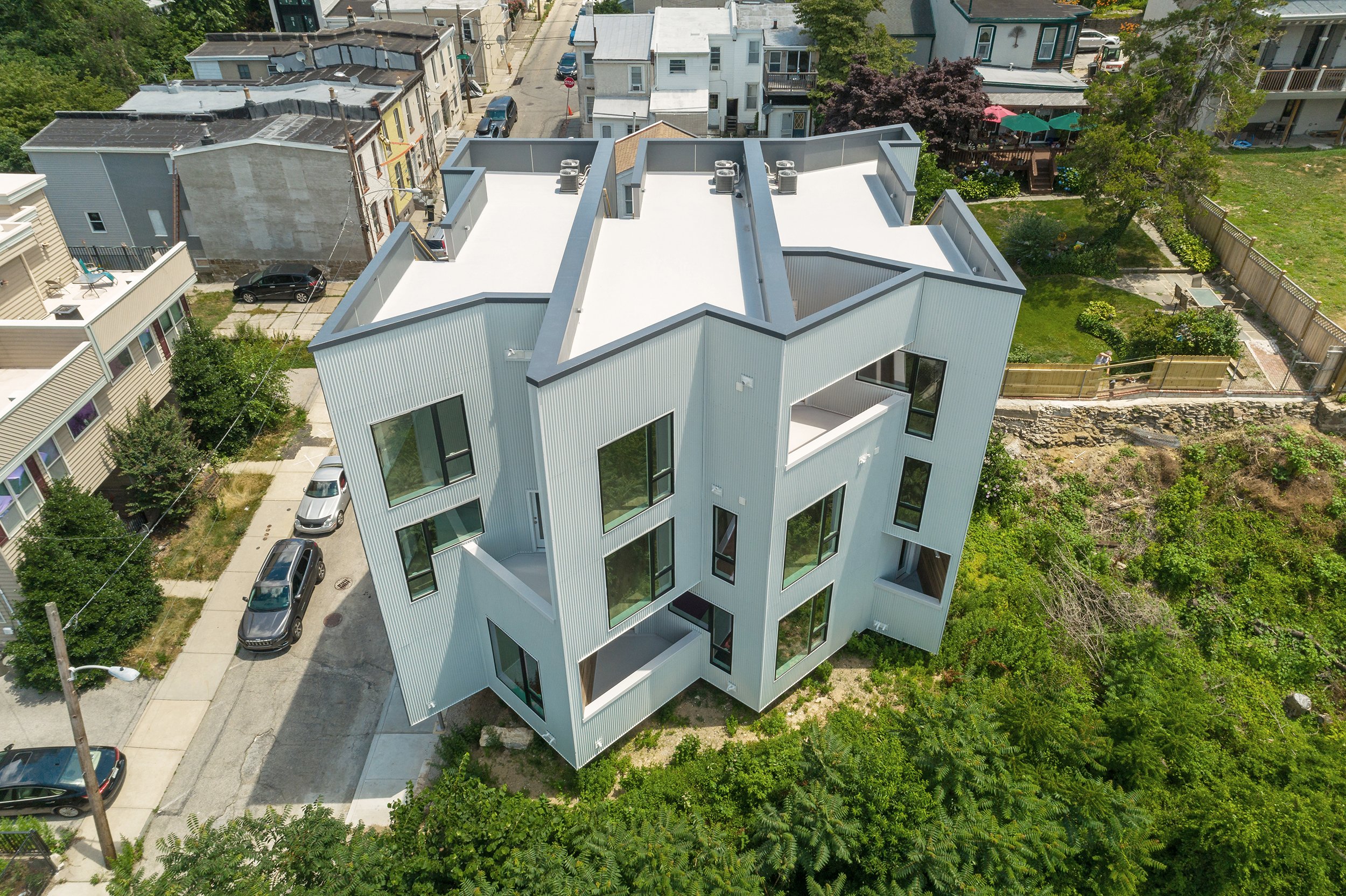The image captures a vibrant outdoor daytime scene taken from approximately seven or eight stories above ground. The full-color photograph features a detailed view of a residential neighborhood below. In the lower right segment and spanning most of the bottom, a dense cluster of trees creates a lush green foreground, partially enclosed by a wooden fence. 

Dominating the central part of the scene is a uniquely designed three-story apartment building, characterized by its modern, angular architecture. The white structure stands out with zig-zagging corners and numerous hard aesthetic lines, giving it a futuristic vibe. The building’s flat roofs are equipped with drainage solutions, and visible stairways suggest access to the roof for recreational purposes. Air conditioning units dot the rooftop, adding to the building’s contemporary feel.

To the left of the building, a street lined with parked cars weaves through the neighborhood. Additional apartment buildings and homes line the street, and power lines stretch across the upper left corner of the image, hinting at the urban setting. In the background, more residential structures are visible, nestled among trees, contributing to the site’s densely populated yet nature-integrated atmosphere.